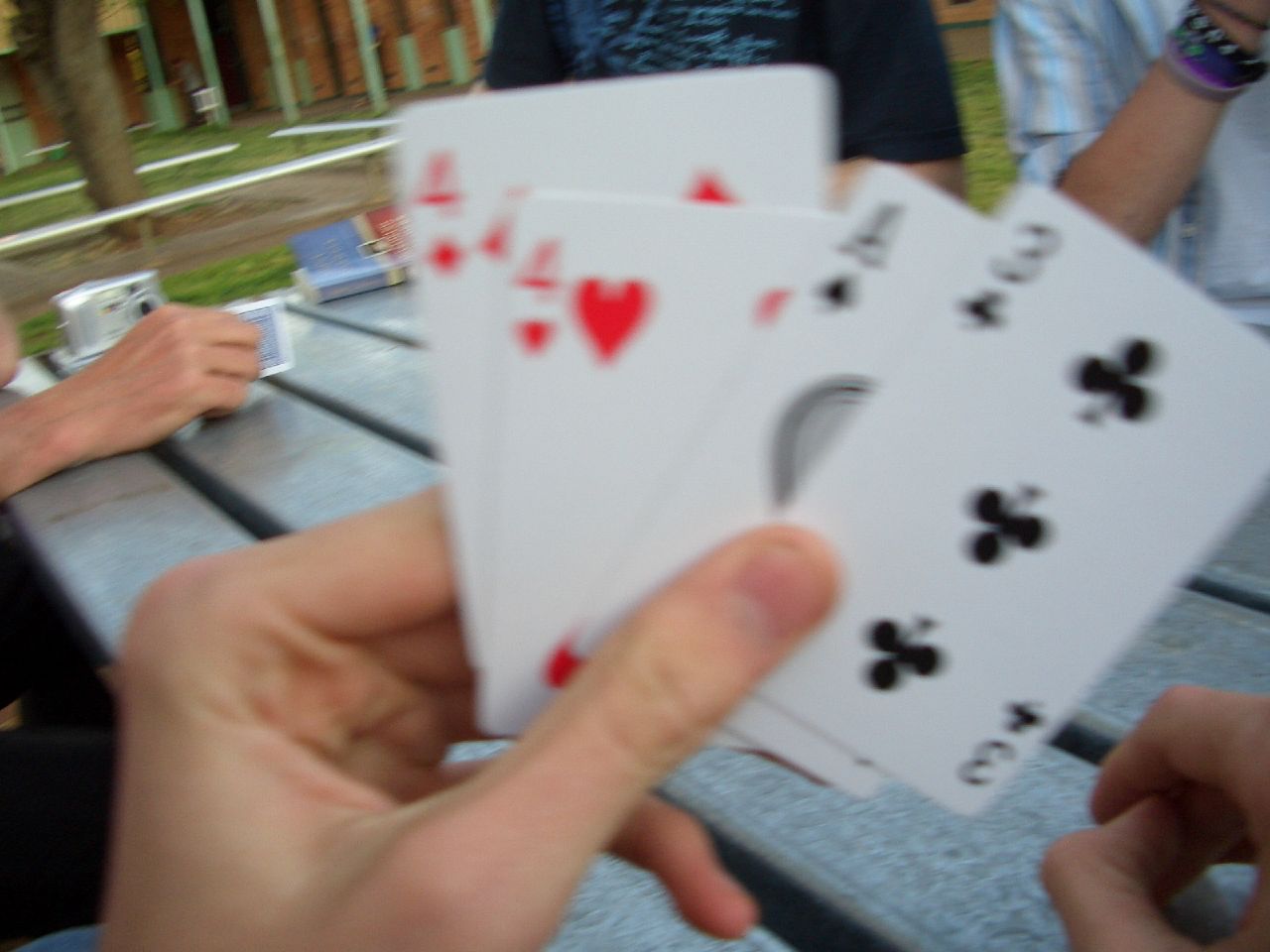A group of four young students are sitting at a wooden picnic bench, engrossed in a game of cards. The scene appears to be set on school grounds, with verdant surroundings and buildings visible in the background. A large tree, encircled with protective railings likely to prevent students from climbing, stands prominently nearby, reinforcing the educational nature of the setting.

At the table, visible on one side is a student whose hand is partially captured, tightly holding his cards. An old digital camera rests on the bench just beyond his hand. Opposite him sits another student dressed in a dark blue shirt with a turquoise script, though the text is indistinct due to blurriness. The person closest to the photographer reveals their hand, holding a four of diamonds, four of hearts, ace of spades, and three of clubs. Directly across from them is a student wearing a shirt, his wrist adorned with numerous friendship bracelets and beads, adding a touch of individuality to the group dynamic.